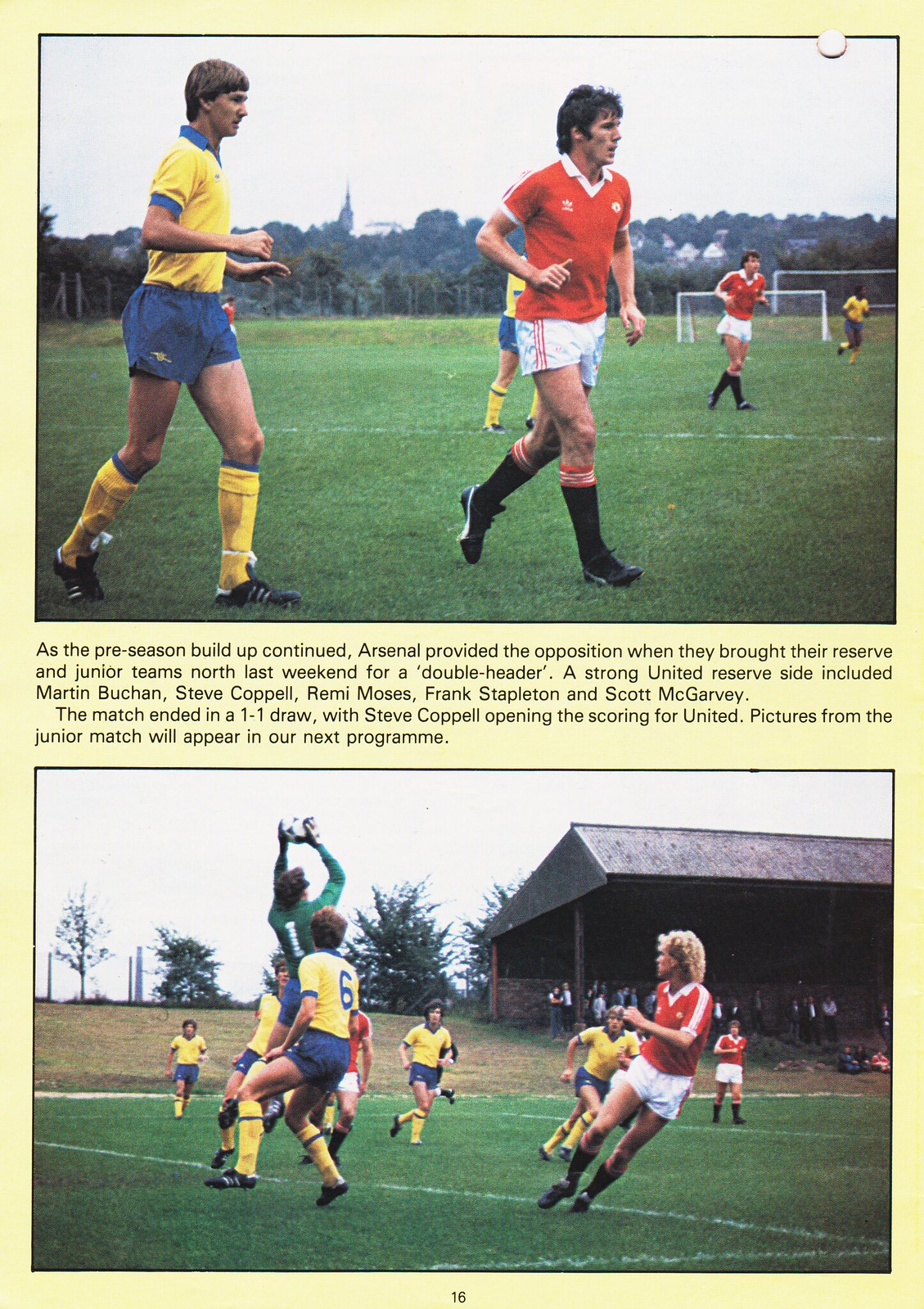The image is a page from a game day program or magazine with a yellow background, featuring two small photos bordered in black. At the top, a picture shows a soccer game with several players, some in yellow and blue uniforms and others in red and white, moving quickly across the green playing field. Among the players, one in a yellow and blue uniform is prominently positioned near another player in a red and white uniform, with some additional players further back and a goalpost visible in the rear. Below this, the second photo captures the action in full motion: a player wearing green leaps into the air with his arms outstretched, holding a soccer ball as a hopeful player in yellow and blue reaches for it. Several other yellow and blue uniformed players approach from behind, while a red and white player moves quickly in the foreground, and another red and white player is further back, with a barn-like structure in the distance. The center of the page contains text that reads, “As the preseason buildup continued, Arsenal provided the opposition when they brought their reserve and junior teams north last weekend for a doubleheader. A strong United reserve side included Martin Buchan, Steve Koppel, Remy Moses, Frank Stapleton, and Scott McGarvey. The match ended in a one-to-one draw with Steve Koppel opening the scoring for United. Pictures from the junior match will appear in our next program.” The page is numbered 16 in black font at the bottom.